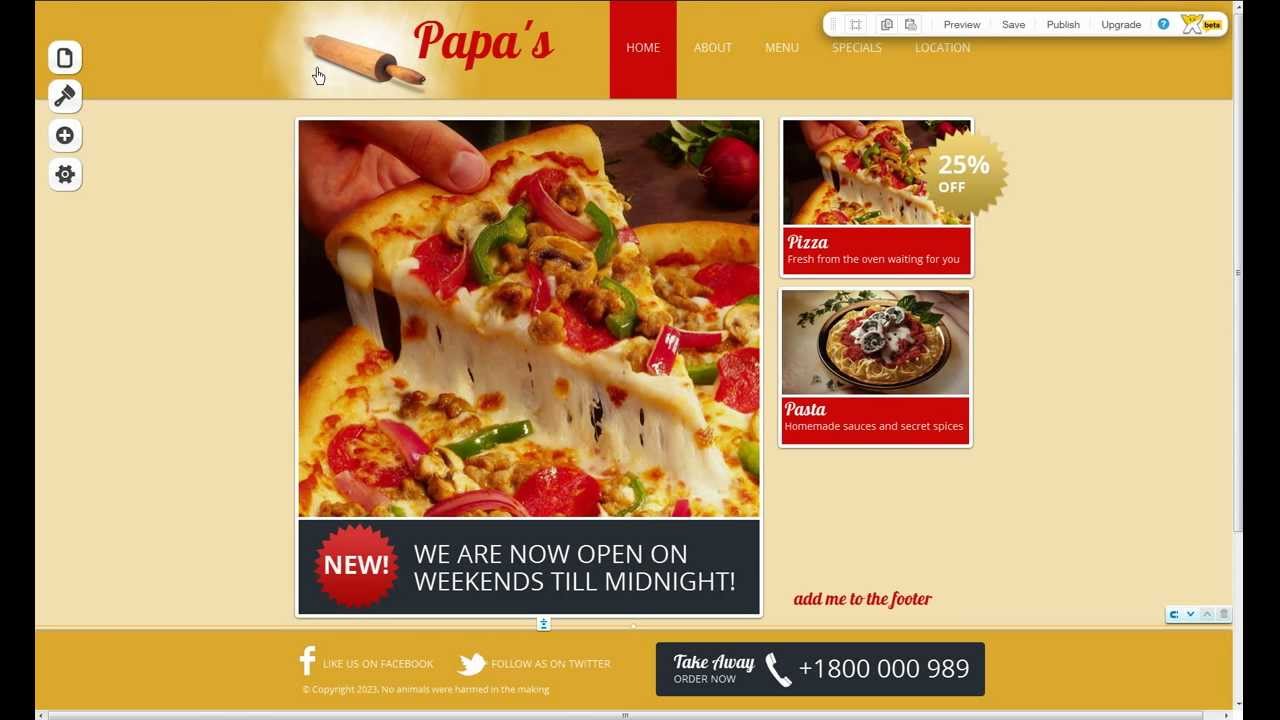Caption for the image:

At Papa's Pizza Joint, the warm and inviting logo features a rolling pin and "Papa's" in an orange box, accompanied by navigation links: Home, About, Menu, Specials, and Locator. Below this, an enticing image showcases a delicious pizza slice, laden with sausage, green and red peppers, onions, mushrooms, pepperoni, and a generous amount of melted cheese stretching from the adjacent slices. Prominently, a banner announces, "New: We are now open on weekends till midnight." There's also a special offer indicating that pizzas are now 25% off, served fresh from the oven. Additionally, Papa's offers authentic pasta dishes made with sausage and secret spices. Don't miss the footer which includes the takeaway order number for convenient menu orders.